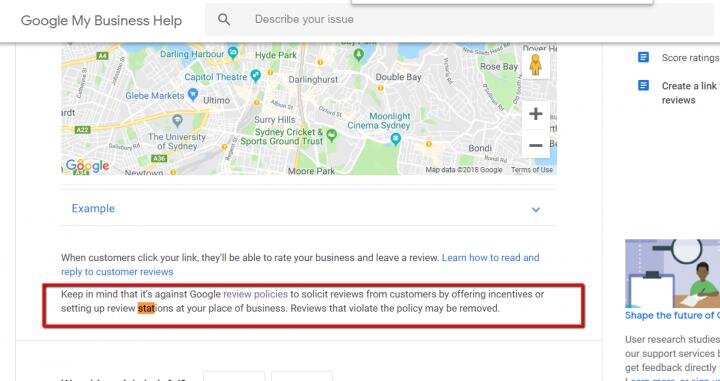This image is a detailed screenshot related to "Google My Business Help" aimed at assisting business owners in managing their online presence and reviews. The main interface features a central search bar at the top labeled "Describe Your Issue," encouraging users to input specific issues they need help with.

A map of Sydney, Australia, occupies the central part of the image, highlighting notable locations such as Moonlight Cinema Sydney, Sydney Cricket and Sports Ground Trust, The University of Sydney, Globe Market, Darling Harbour, Hyde Park, Double Bay, and Rose Bay. Bondi is also prominently marked. The map includes zoom controls (plus and minus) and a draggable little person icon for street view functionality.

To the right of the map, there is a section titled "Score Ratings and Create a Link," under which an example drop-down menu is visible. This section explains that when customers click a provided link, they will be able to rate the business and leave a review. A cautionary note advises business owners that soliciting reviews through incentives or setting up review stations at their business location is against Google review policies, and such reviews may be removed if they violate these terms. Business owners are also guided on how to read and reply to customer reviews.

A glitch is noted where the recording timer on the interface has become unresponsive, stuck and surpassing the intended duration, currently displayed at 1 minute and 45 seconds.

Overall, the image provides a comprehensive look at the tools and guidelines available to business owners for managing their Google My Business reviews, ensuring compliance with Google’s policies, and enhancing customer engagement through feedback.